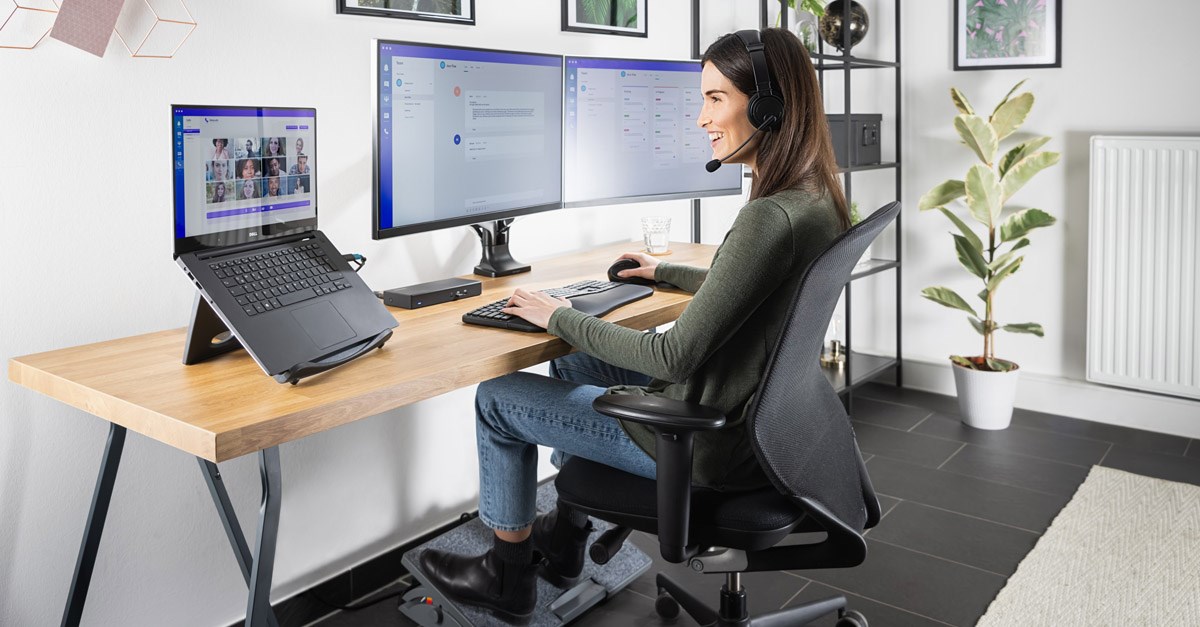The image depicts a woman with a fair complexion and dark brown shoulder-length hair, sitting in a modern, minimalist home office. She is dressed in blue jeans, black boots, and a dark green long-sleeve top. The woman is smiling as she looks to her left, engaged in a remote office meeting or Zoom call, evidenced by the black headset with a microphone she is wearing. Her feet are elevated on a gray adjustable footrest, indicating comfort and ergonomics are important to her workspace.

In front of her is a large wooden desk with black legs, supporting a setup of dual curved monitors positioned to her right and a laptop perched on a stand to her left. The laptop screen displays participants of the virtual meeting. She appears to be actively participating, with her hands placed on a keyboard and mouse.

The room is characterized by white walls adorned with several black-framed pictures, depicting nature scenes like leaves and branches. The flooring is a combination of black tile and a cream-colored carpet behind her. To the right of her desk stands a tall green plant in a white pot, about three feet high, and a white baseboard heater that blends into the wall. There is also a cube-style black shelf in the corner, holding various knickknacks including a black marble globe and a small black box, lending an industrial yet cozy feel to her home office environment.